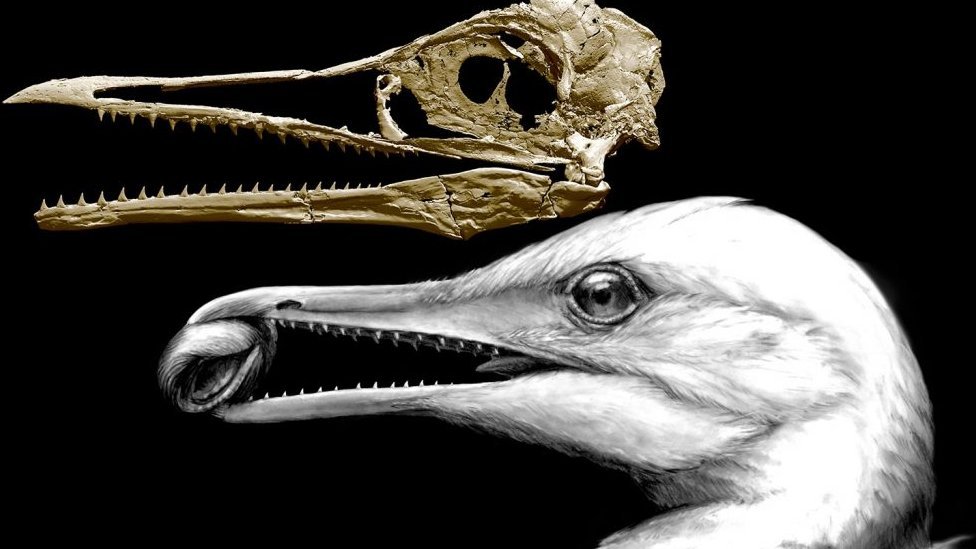This image appears to be a diagram from a textbook, featuring a detailed composition of a bird on a black background. The main focus is a white bird with short white plush feathers, a dark beady eye, and a long, narrow beak that is slightly open, revealing small teeth and a short tongue. The bird is depicted holding an object, likely a pistachio shell, at the edge of its beak. Directly above, a skeletal view of the same bird is displayed, showing the bone structure with an open beak, emphasizing the teeth and hollow eye socket. The dual representation of the bird, both in its feathered form and as a skeleton, highlights the anatomical details and structure, providing a comprehensive visual relationship between the external appearance and internal skeleton.